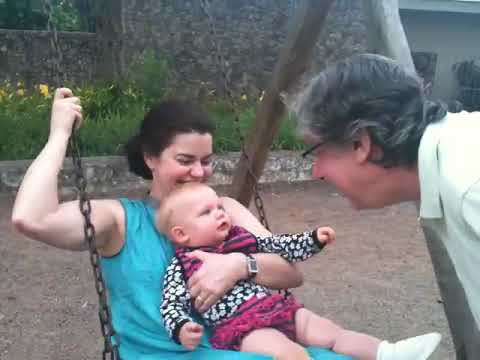In this color photograph, oriented in landscape, a young mother sits on a sturdy chain swing set, holding a baby on her lap. The woman, placed prominently in the foreground, has dark brown hair pulled back into a ponytail and is dressed in a sleeveless blue tank top. Her right hand grips one of the swing's chains for support, while her left arm lovingly cradles the baby. The little one, around nine months to a year old, sports short blonde hair and a happy expression directed at a man beside them. The baby is clad in a long-sleeve black and white shirt adorned with purple and black stripes, a bib, red and pink diaper pants, and white shoes.

The man, possibly the baby’s grandfather, is leaning in from the right, engaging the baby with a warm smile. He has gray hair and wears black glasses, a long-sleeve white button-down shirt, and a tie, paired with shorts. He appears thoroughly fascinated by the baby’s expressions.

The backdrop of this idyllic scene features a gray and brown brick house with a garage door, partially obscured behind a short stone retaining wall. Between the wall and the house, tall green plants with yellow flowers add a touch of natural beauty. The swing set is supported by a robust wooden crisscrossed frame, while the ground beneath is a simple expanse of brown dirt, enhancing the scene’s rustic charm.

This image, captured with a slight blurriness, evokes a moment of tender family interaction and joy.